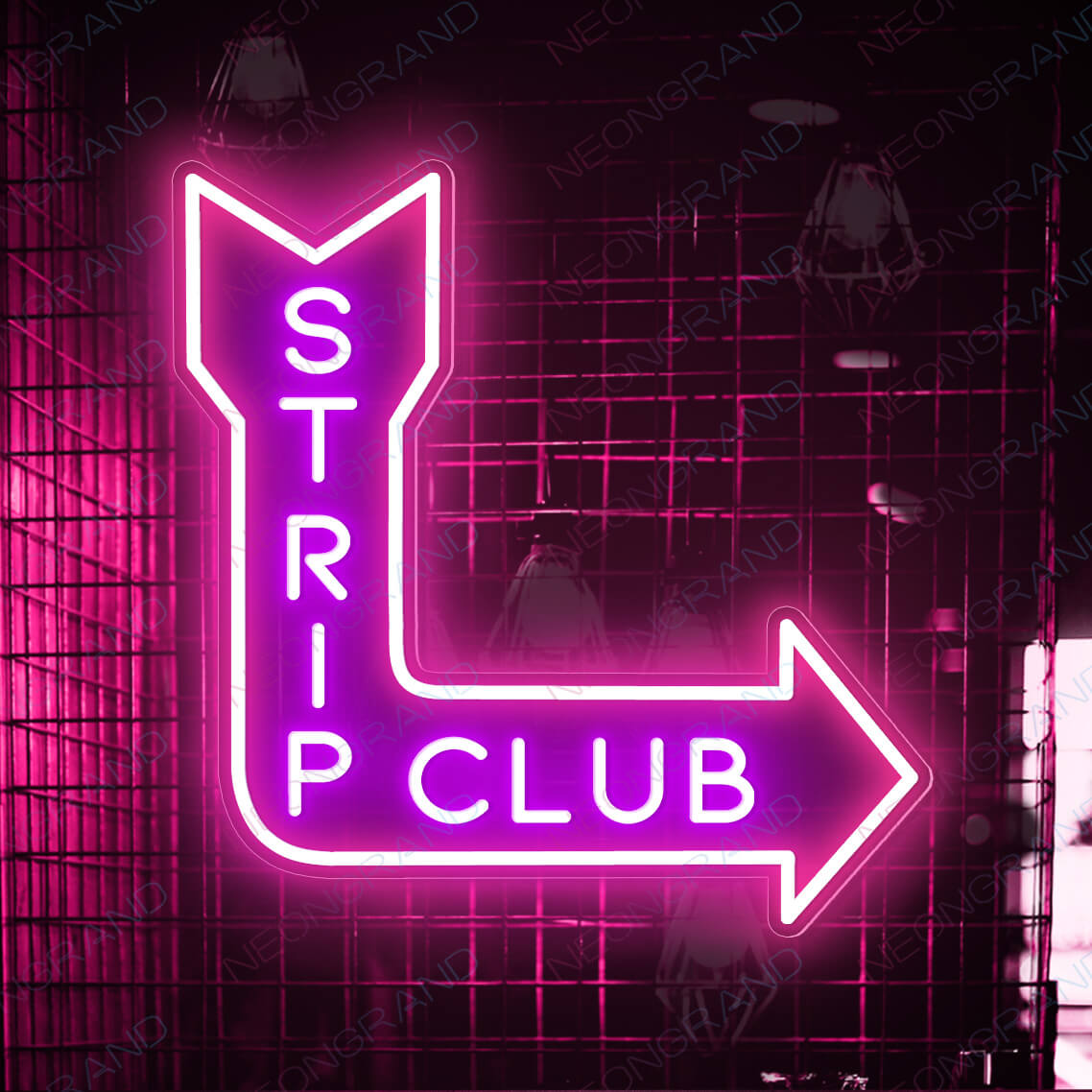The image captures a vibrant neon sign fixed to a metal grid fence, clearly indicating a strip club. The sign is designed as an arrow that starts vertically from the top left, bends 90 degrees to the right, and finishes with an arrowhead. The word "strip" is written vertically along the descending part of the arrow, while "club" is displayed horizontally along the rightward extension. The neon lights emit a luminous pink or purplish glow, creating a striking contrast against the dark metal fence and the shadowy background. Although there are additional lamps visible in the scene, they remain unlit, adding a hint of depth with their faint outlines and bulb details. Notably, the image is watermarked with the brand name "Neon Brand" without obscuring the neon sign itself. In the bottom right corner, a partially visible door or window adds a subtle, unfinished element to the composition.